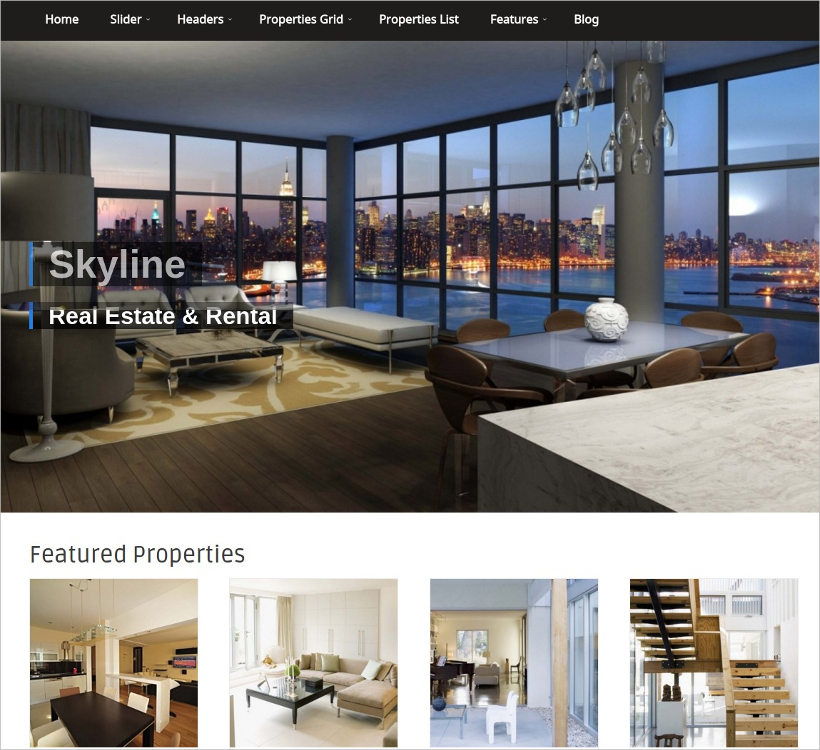This image captures a screenshot of a sophisticated real estate and rental website, likely named "Skyline Real Estate and Rental," based on the partially visible text beneath an opaque mask. The website's navigation bar, rendered in thin black with white text, runs across the top, featuring clickable sections such as Home, Slider, Headers, Properties Grid, Properties List, Features, and Blog.

Dominating the page below the navigation bar is a high-resolution image of a luxurious waterfront apartment or house. The focal point is a spacious living room, boasting a wall entirely composed of floor-to-ceiling windows that afford a breathtaking view of a harbor and city skyline. The interior exudes elegance, with its polished wood flooring, chic furniture, and champagne glasses suspended from the ceiling. It epitomizes high-end urban living.

Beneath this striking image, in a crisp white section, the website showcases "Featured Properties." This section includes four square images, each depicting similarly upscale properties, hinting at the exclusivity and luxury the website offers.